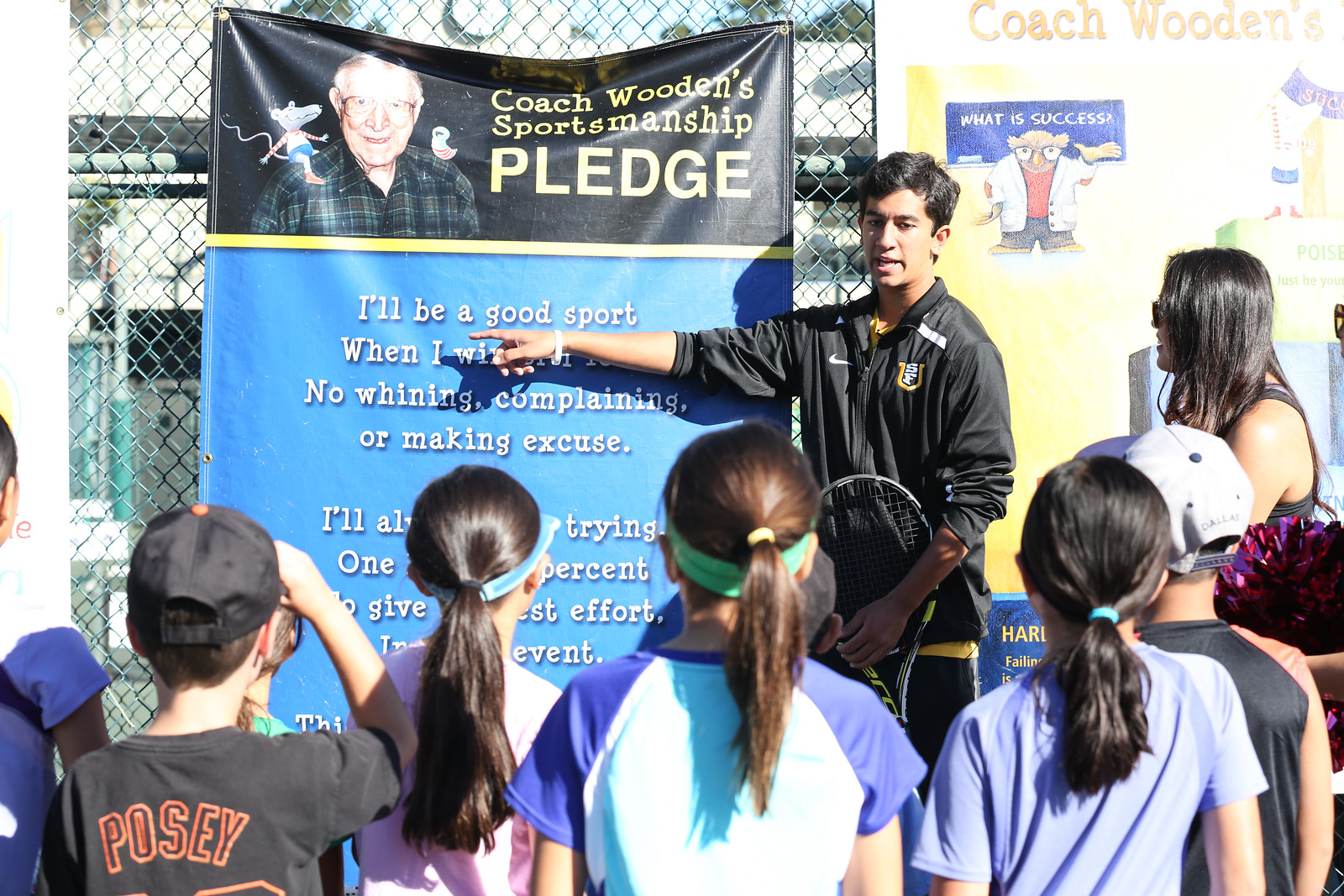In this outdoor photo, a group of children, mostly girls with ponytails wearing blue and white short-sleeved shirts, stand facing a man with short dark hair and a black jacket. The man, holding a tennis racket, points at a sign attached to a chain-link fence. The sign, titled "Coach Wooden Sportsmanship Pledge," starts with "I'll be a good sport" and includes phrases like "no whining, complaining, or making excuses." Some text on the sign is obscured by the man's arm and a girl's head. To the right of the man, a woman with brown hair in a tank top and sunglasses watches. The setting suggests a sporting event, possibly a tennis practice or lesson.